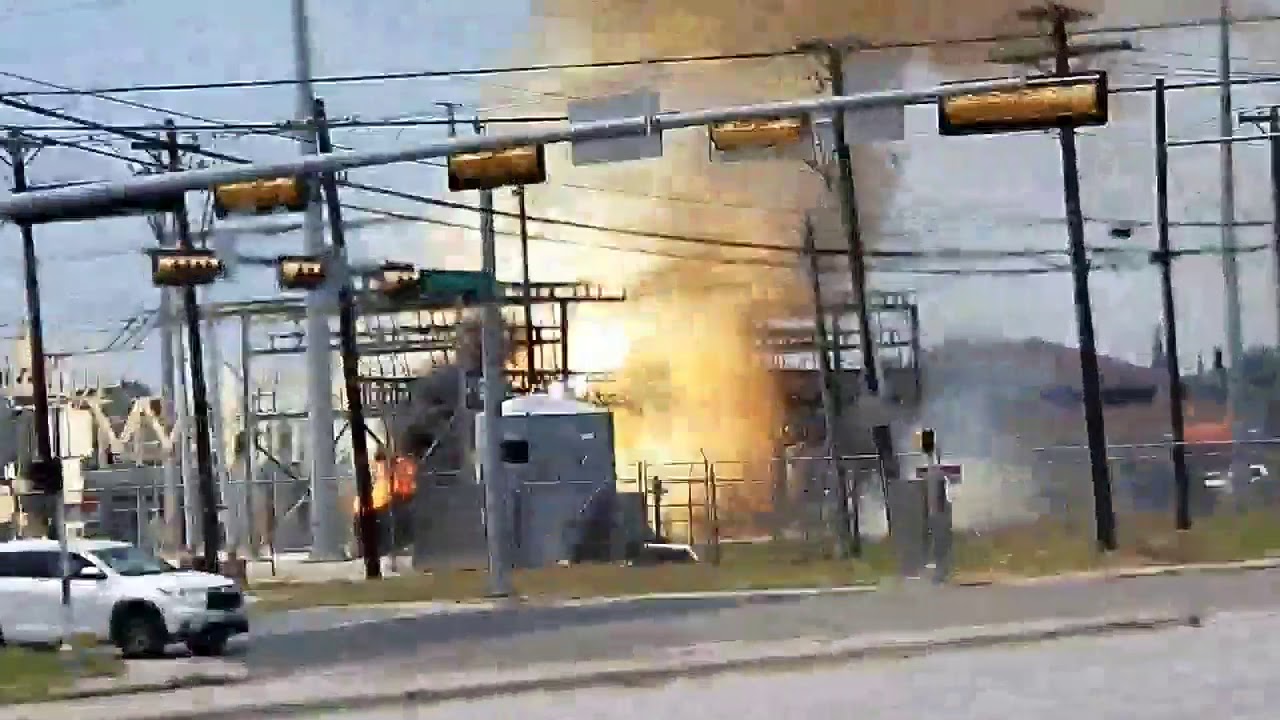The image depicts a blurry, CCTV-style footage of a chaotic scene at an intersection near a power facility that appears to have suffered an explosion or fire. A white car, likely an SUV, is stopped at a traffic light or stop sign in the foreground. The scene in the background is dominated by a large burst of dust, smoke, and flames, rising dramatically from behind a fenced area containing an electrical transformer or power plant. The explosion site is characterized by gray structures, power lines, and telephone poles, with bright yellow and orange flames suggesting a severe fire possibly caused by a recent small explosion or a lightning strike. The building in the distance is obscured by thick smoke, adding to the overall sense of disaster and confusion in the image. The sky is blue, contrasting starkly with the chaotic foreground, and the ground is a medium gray, consistent with the CCTV footage style capturing the scene.